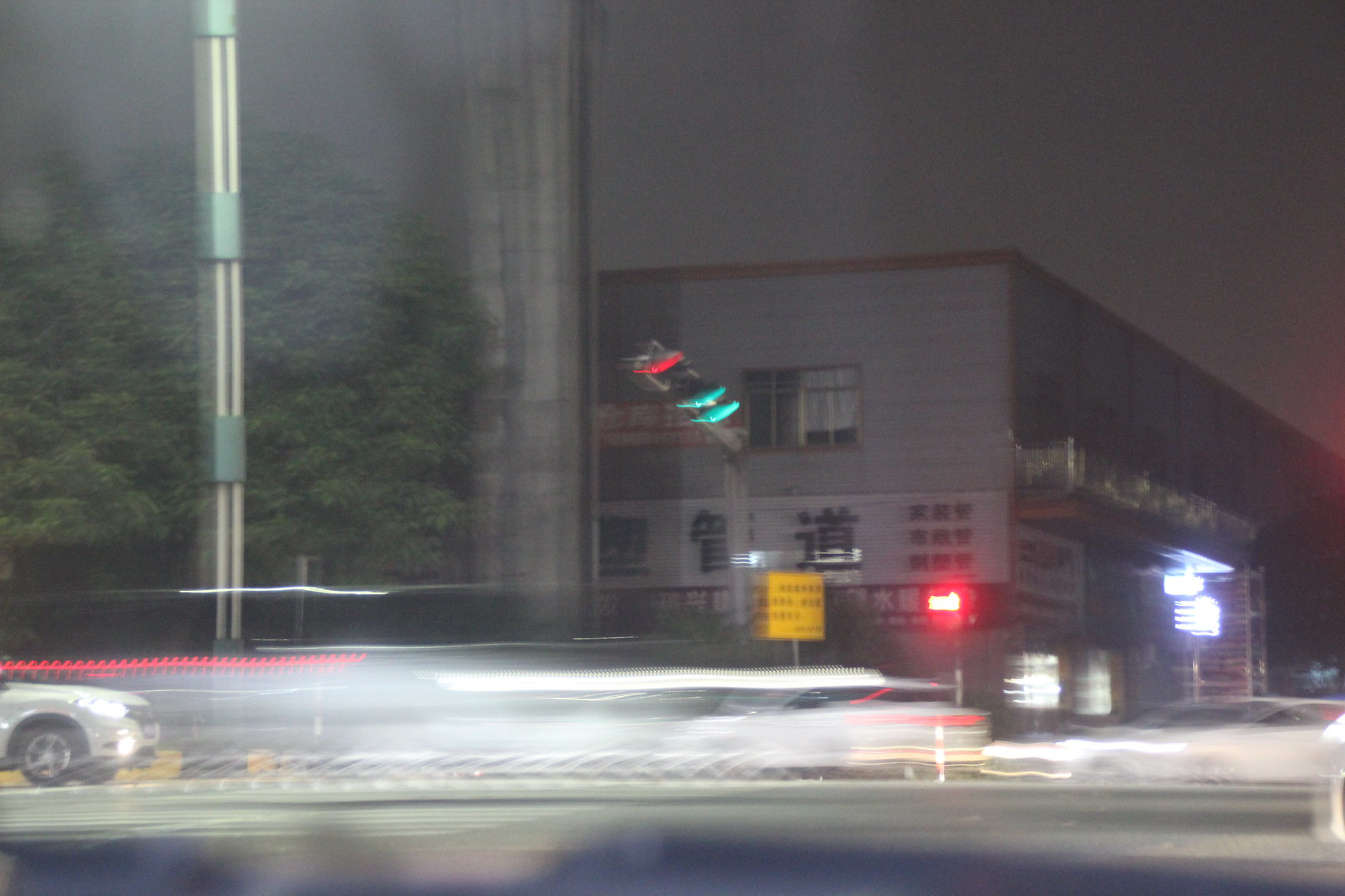This nighttime, high-speed photograph captures an urban street scene filled with dynamic motion. Taken across the street from a gray building with large, visible windows, the image showcases a car zooming by at such speed that its form is heavily motion-blurred. The action unfolds under multiple street lights, including a prominently visible traffic light displaying a green signal, indicating the car is speeding through an intersection. On the upper left-hand corner, a large tree provides some contrasting stillness to the bustling scene. Additionally, a single white car can be observed on the right side of the image, albeit also blurred due to its high speed. The overall setting seems desolate, with no foot traffic and an industrial feel suggested by the building's utilitarian design. The blend of artificial lights and motion-blur create a captivating sense of urgency and movement in this snapshot of urban nightlife.